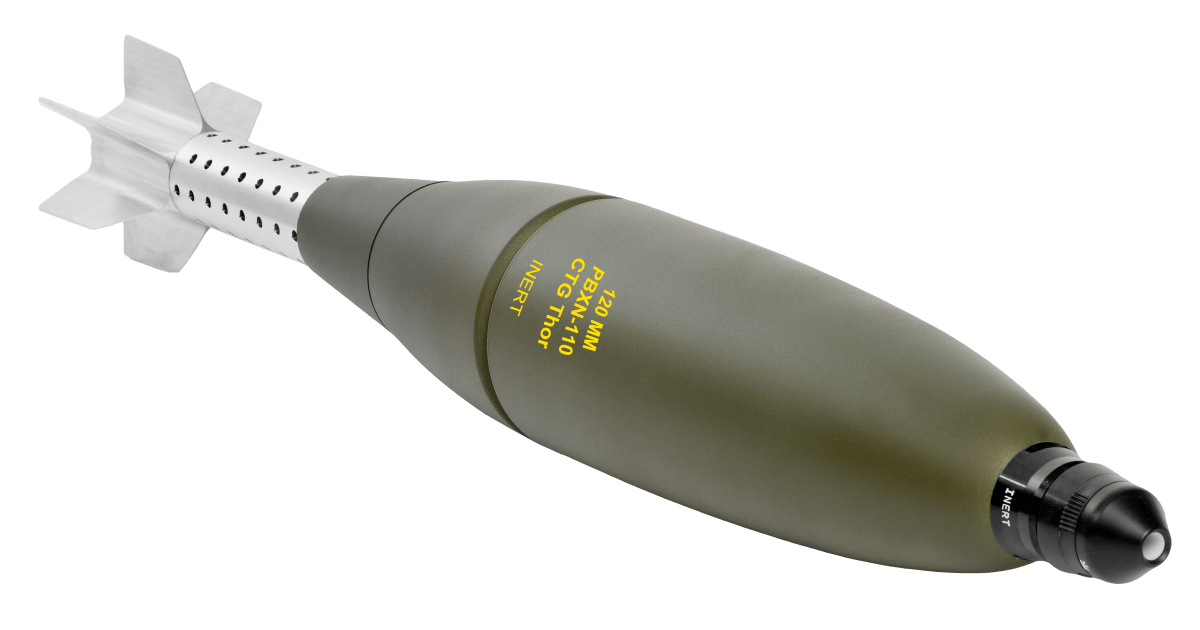This image showcases an inert military weapon with no background, isolated against a white backdrop. The weapon appears in a very dark olive green color, tapering to a black tip at the front. Yellow text located on the front of the body reads "120mm PBXN-110 CTG Thor inert," indicating its inert status and specifying its model. The text stands out vividly against the dark backdrop. The missile-like object, possibly a torpedo or bomb, transitions from its dark green main body to a silver tail section. This tail section features around six small guidance fins, evenly arranged and interspersed with tiny black holes. The object is positioned centrally in the frame, extending from the top left to the bottom right, displaying a smooth, oval shape and a detailed construction that emphasizes its intricate design and intended aerodynamics.